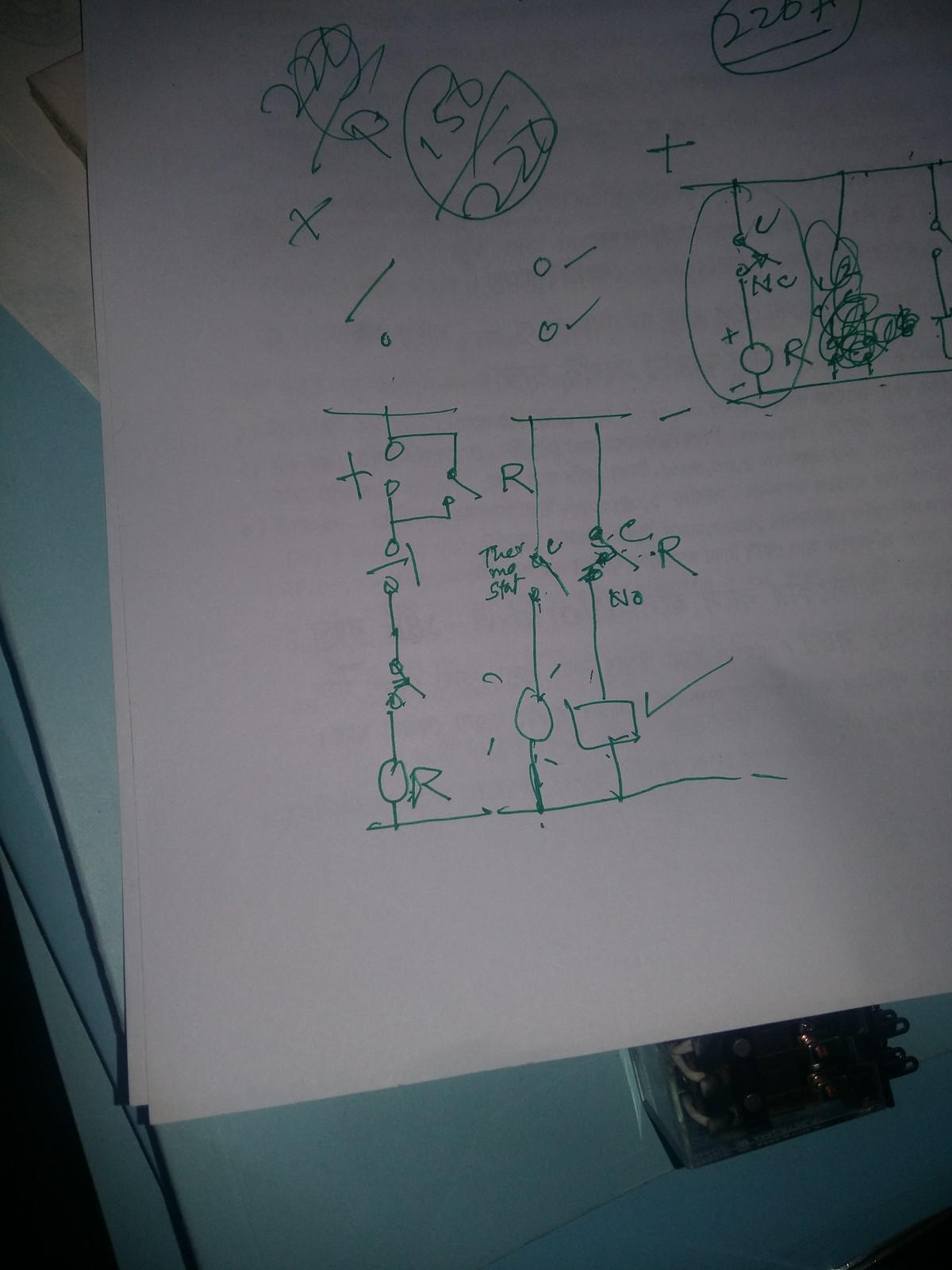The image depicts a hand-drawn formulation on a white piece of paper using a green pen. At the top, there are various numbers, with "150 over 220" prominently displayed and crossed off. The area is also interspersed with Xs, check marks, and zeros marked with check marks next to them. 

Moving towards the center, there's a complex arrangement of lines and circles: a descending line terminating in an "O," followed by another line that leads to yet another "O." This pattern repeats several times. Specifically, there is a plus sign between two of the "O" elements, indicating an equation. This sequence concludes with an "O" followed by an equal sign and another "O," which is crossed off. 

Below this, a larger "O" is accompanied by the letter "R." Above this detailed section, another delineation shows lines descending into the letters "R" and "C" on opposite sides. 

Further down, there's a cryptic note saying "there no stat," leading into another sequence of lines and "O" shapes. Finally, there's a line terminating in a square, which has a check mark beside it, signifying completion or verification.

This detailed formulation suggests a mix of mathematical notation and possibly experimental data or a flowchart, all intricately composed by hand.